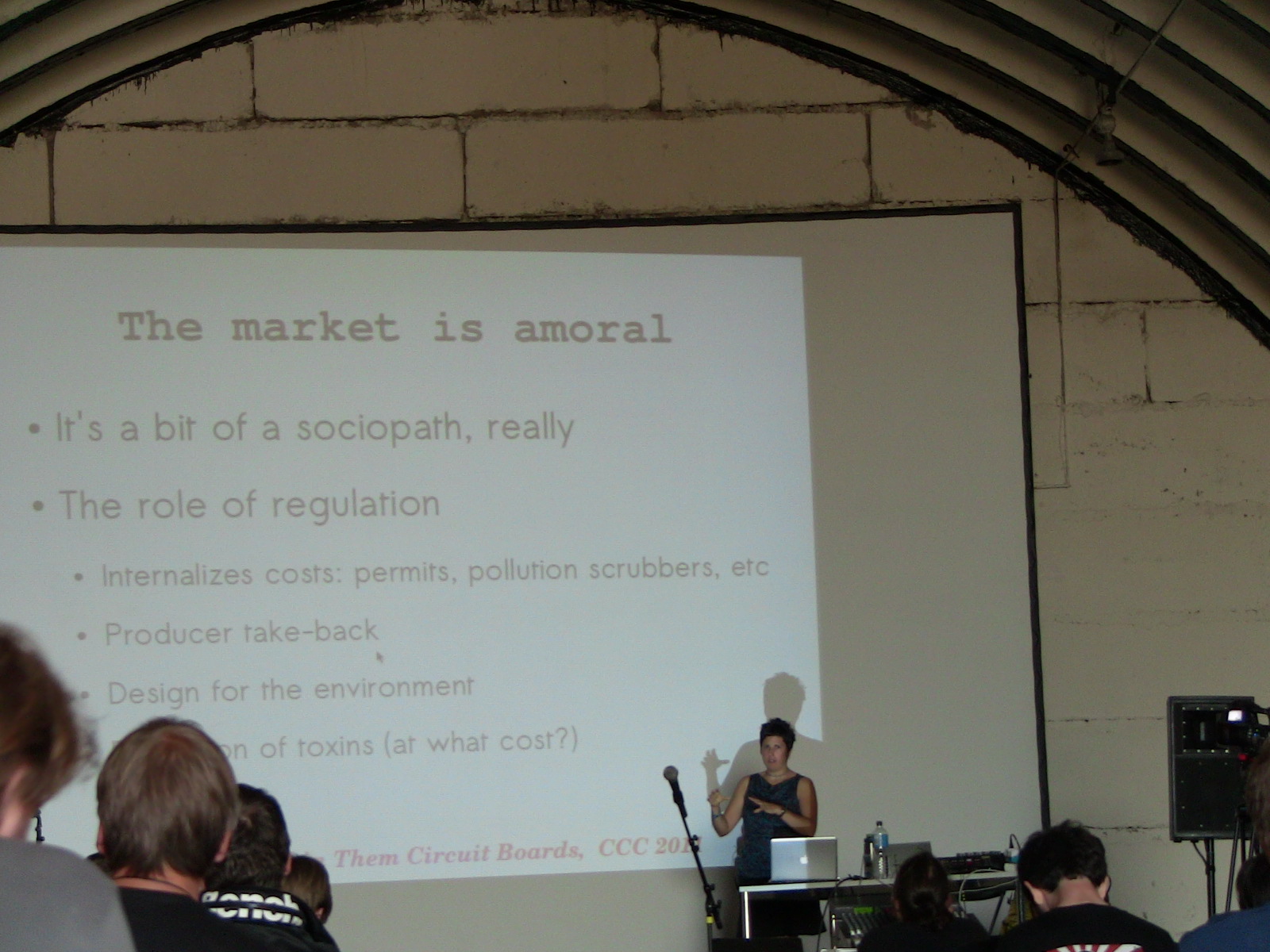The image captures a business seminar taking place inside a lecture hall with a distinct architectural design featuring long horizontal brick patterns on the walls and semicircular wavy patterns on the ceiling. Several audience members, visible only from the back, are seated facing a large projection screen. At the front of the hall, a young woman with short black hair, dressed in a sleeveless top, stands behind a microphone, giving a presentation. On the desk in front of her, alongside a water bottle and some equipment, is an Apple Mac laptop. The projected slide on the screen is titled "The Market is Amoral" and includes bullet points such as "It's a bit of a sociopath, really," "The role of regulation," "Internalizes costs," "Permits," "Pollution scrubbers, etc.," "Producer take-back," and "Designed for the environment." Some additional text is partially obscured by one of the audience members' heads and a microphone stand, including phrases about toxins and a footnote that mentions "circuit boards, CCC 2000." The environment suggests an engaged audience attentively listening to the detailed exposition provided by the speaker.